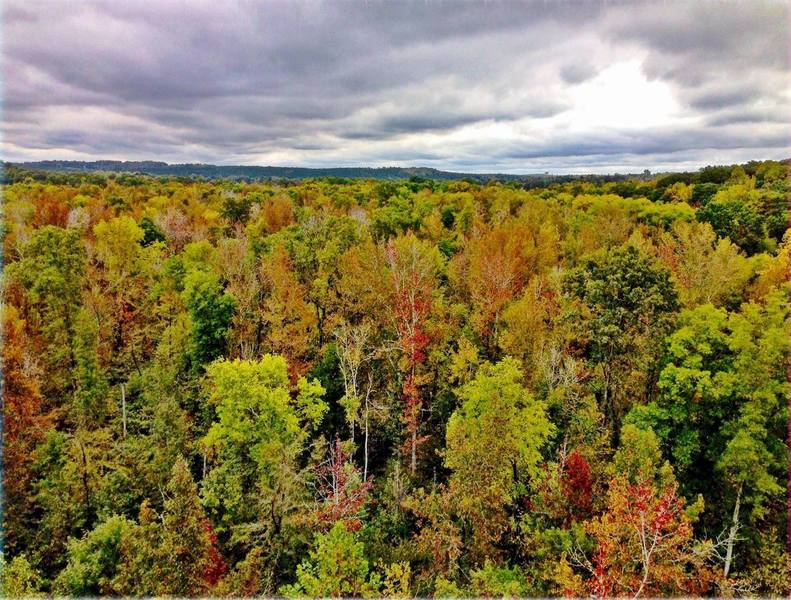The image captures a densely packed forest viewed from an elevated vantage point, possibly a tall building, looking across a sea of treetops. The scene suggests the onset of fall as a variety of colors—green, orange, yellow, red, and brown—intermix among the foliage. At the bottom center-right, a tree with striking red and orange branches stands out, accompanied by smaller trees with red leaves nearby. Two slender trees with sparse foliage are positioned centrally. The left side predominantly features green mixed with some orange, whereas the right side shows a majority of green hues. The dense forest extends into the distance, showcasing a tapestry of green, orange, yellow, and even some white-tipped trees. A distant, indistinct horizon lies further back, possibly delineating a less densely treed area. Above, a predominantly gray sky looms, laden with clouds except for a small, almost triangular patch of clear sky at the top right corner. Enhancing the natural beauty, a mountain range can be seen in the background, rising above the forest and also speckled with autumnal colors. Overall, the image beautifully captures the diverse palette and serenity of a forest transitioning into fall.